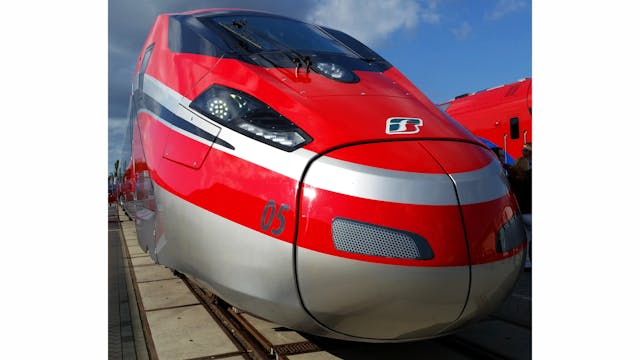The photograph captures the front of a sleek, modern electric train, predominantly fire engine red with metallic gray and black accents. The train's nose, reminiscent of a snake's head, features a slub-nosed design with a prominent number "05" displayed in bold text. At the very front, there's a red and blue letter "B" logo, accompanied by smaller blue, red, and white details which add to its striking appearance. The train is set against a backdrop of a clear blue sky with scattered white clouds, indicating a sunny midday. The image, taken from a frontal angle, shows the train on its tracks, with another red train visible to the right side. The train's large, flat, and sleek black window area, surrounded by a silver-gray hood equipped with a grill and windscreen wipers, adds a touch of modern efficiency to its design. In the lower part of the frame, train sidings and rails are visible, giving context to the train's environment. The overall composition emphasizes the train's dynamic and robust look.